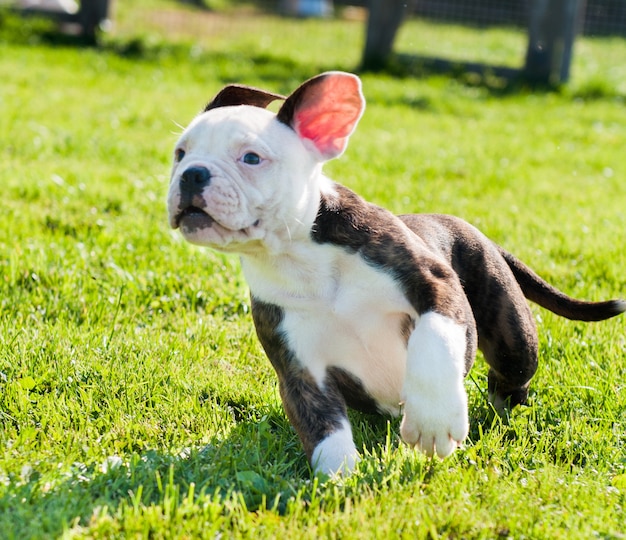In this vibrant photo, a small puppy, potentially a French Bulldog or Bull Terrier mix, is captured mid-run across a lush expanse of green grass on a sunny day. The puppy exhibits a playful energy, with its ears blown back by the wind, showcasing the pink interior of one ear. It appears to be around two to three months old and is predominantly white with distinctive brown patches on its body. The pup's white face, chest, and front paws contrast against its brown tail, which is visible on the right-hand side of the image. His dark brown eyes and black nose stand out, with a touch of black below the nose and mouth adding character to his expression. The photo features the puppy's shadow stretching towards the lower left corner, and while there are indistinct figures in the background, the focus remains entirely on the joyous puppy, making it the undeniable centerpiece of this charming scene.